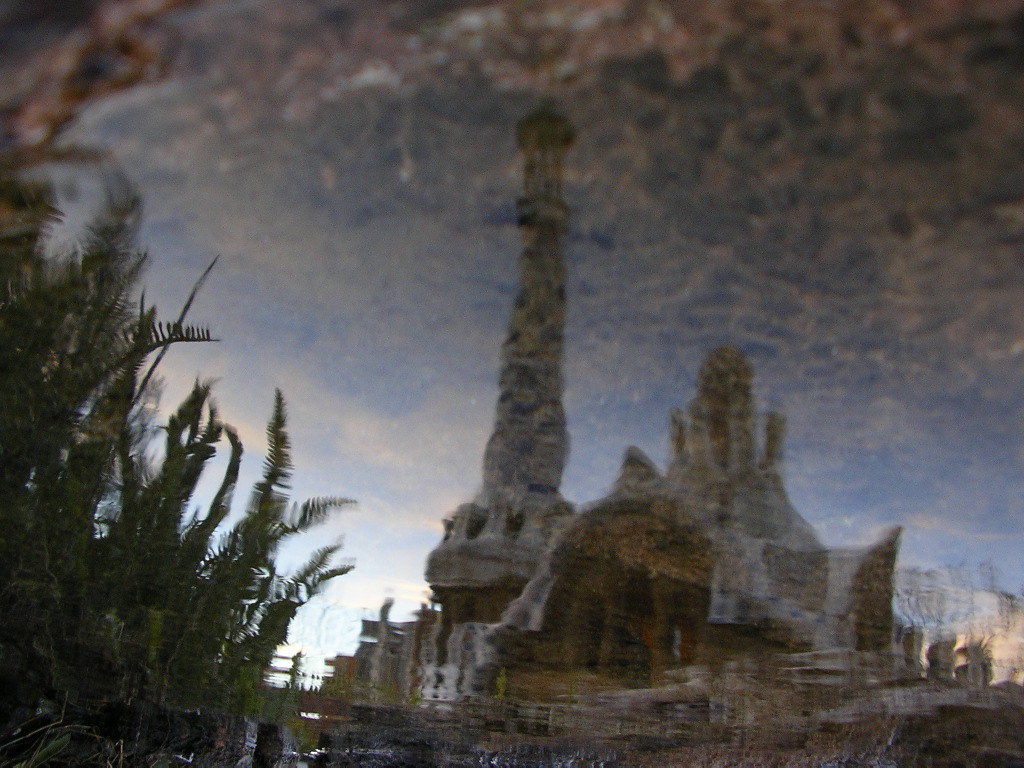This image captures a city skyline with an intriguing blend of modern and ancient architectural designs. The composition features a prominent center dominated by a tall, cylindrical building that tapers at the top, adorned with a striking blue, spiky detail. Surrounding this central structure are older, shorter buildings of varying styles, with colors ranging from light blue and green to gray, brown, and tan. 

In the bottom left corner, there's a green plant consisting of tall, skinny stalks with tiny leaves that gradually diminish towards the edges. The sky above is a complex tapestry of blue and grayish clouds, transitioning to a textured pink hue at the top. The lower part of the image appears somewhat distorted, as if viewed through a reflection on water or possibly through a window, adding a surreal, mirrored quality to the scene.

The overall ambiance suggests a moment captured during a time without much direct sunlight, possibly at sunset or sunrise, enhancing the timeless and slightly dreamlike atmosphere of the cityscape.